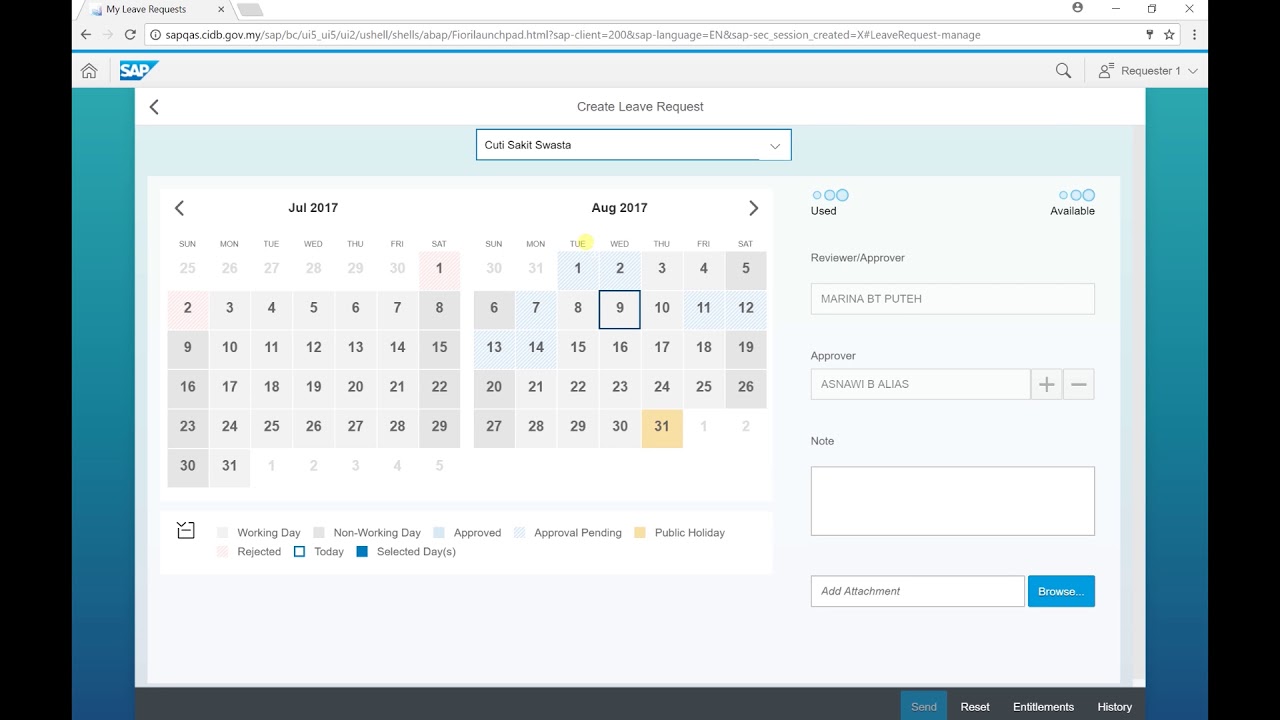This is a screenshot taken from a desktop or laptop computer displaying an interface for managing leave requests within the SAP system. The horizontal image is bordered by thick black rectangles on the left and right sides, while the bottom features a gray bar with various action tabs labeled "Send" (highlighted), "Reset," "Entitlements," and "History." 

At the top, there is a white search bar flanked by essential navigation buttons, including "Go Back," "Go Forward," and "Refresh," as well as icons for "Starring" an item and accessing "More Options." Additional buttons for window control, such as "Minimize," "Full Screen," and "Close," are also present. 

Below the search bar, a tab labeled "My Leave Requests" is visible. The interface shows the SAP logo on a gray background accompanied by a magnifying glass icon for search functionality. There's an option marked "Requester 1" with a dropdown arrow for more options. The section where users can "Create a Leave Request" is presented on a white background with gray text.

In the calendar view, two months are displayed: July 2017 and August 2017. Various dates are boxed or highlighted to indicate public holidays, selected days, and the current day. An area displays leave statistics tagged as "Used" and "Available." Review and approval details show the reviewer as Marina B. T. Puta and the approver as Anzali B. Elias. 

Additionally, there are options to add notes or attachments using plus (+) or minus (–) icons. The text "Curisake Swastika" is also visible, likely indicating the name of the individual logged in or the requestor.